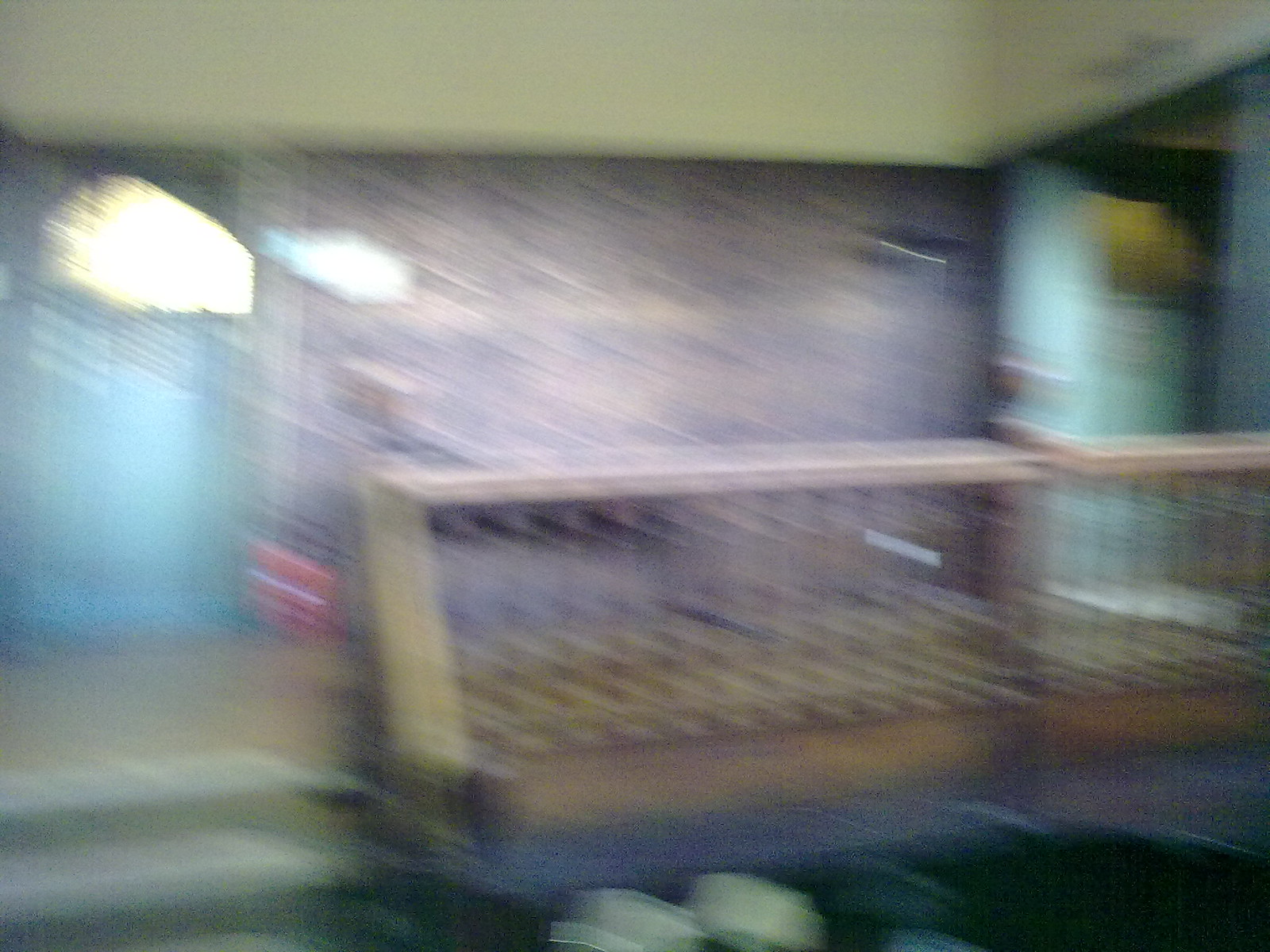This incredibly blurry indoor photograph appears to depict a stair landing with a variety of identifiable elements, despite the significant distortion. Central to the scene is a stairway featuring brown steps, leading upwards to a bluish door that possesses a window above it, influenced by a reflection of light. Adjacent to the stairs is a pale wooden banister stair railing adorned with metal spirals or thin iron rods. The space includes a white or yellowish white ceiling at the top. To the left of the stairway, there is a transition to a lower level, indicated by two steps and a visual play between the wood and metal of the railings. Beyond the steps, there are indistinct glimpses of walls, with one appearing to be a blurry blue and possibly a second door in a robin's egg blue hue. A hallway extends to the right of this stair-landing area, contributing to the distorted and dynamic nature of the image.